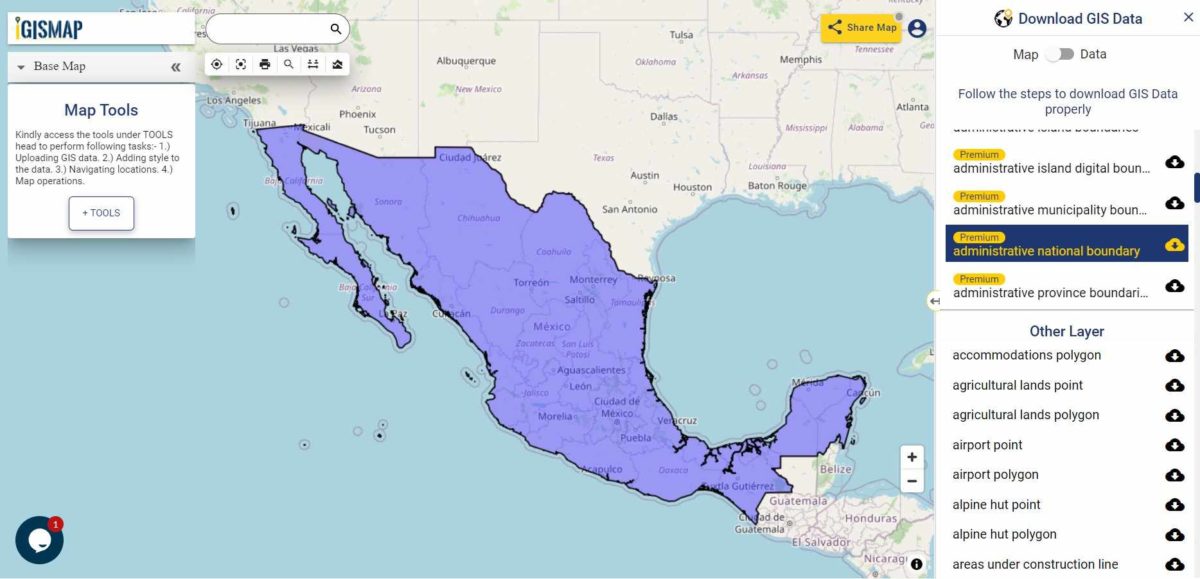A detailed screenshot showcases a GIS map interface focusing on Mexico, which is highlighted in purple, covering the entire country. The lower portion of the United States is also visible at the top of the map, providing a geographical context. The interface includes various map tools, prominently displayed, such as options to "Share Map," and "Download GIS Data." These tools appear multiple times within the screenshot, emphasizing their availability for user interaction.